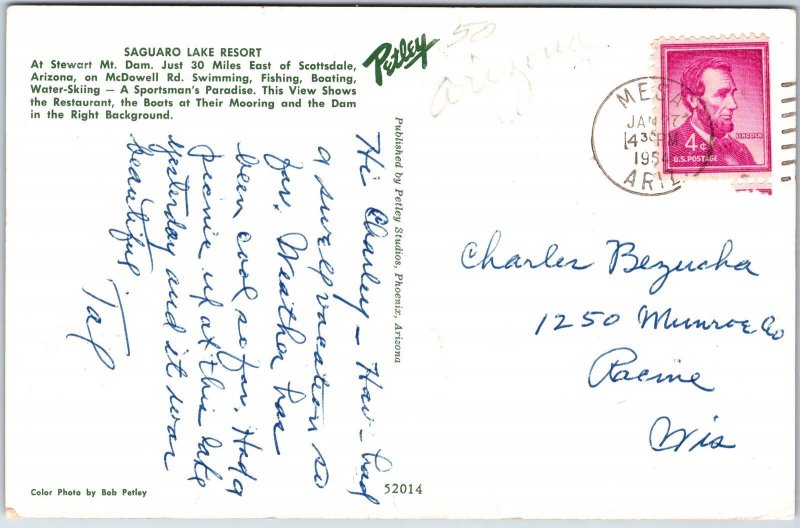The image displays the back of a white postcard that prominently features green cursive text in the top left corner announcing "Saguaro Lake Resort at Stewart Mountain Dam, just 30 miles east of Scottsdale, Arizona on McDowell Road." The text highlights activities such as swimming, fishing, boating, and water skiing, describing it as a sportsman's paradise. The view depicted shows the restaurant, moored boats, and the dam in the right background. Additionally, the upper left section contains the text "Color Photo by Bob Petley" and "Published by Petley Studios, Phoenix, Arizona," along with "Petley" written in green letters. The upper right corner displays a pink 4-cent postage stamp featuring Abraham Lincoln, postmarked January 17, 1954, from Mesa. Addressed to Charles Bazucha at 1215 Monroe, Racine, Wisconsin, the postcard includes a personal note reading, "Hi Charlie. Have had a swell vacation so far. Weather has been cool so far. Had a picnic up at this lake yesterday and it was beautiful." It is signed "TAL."